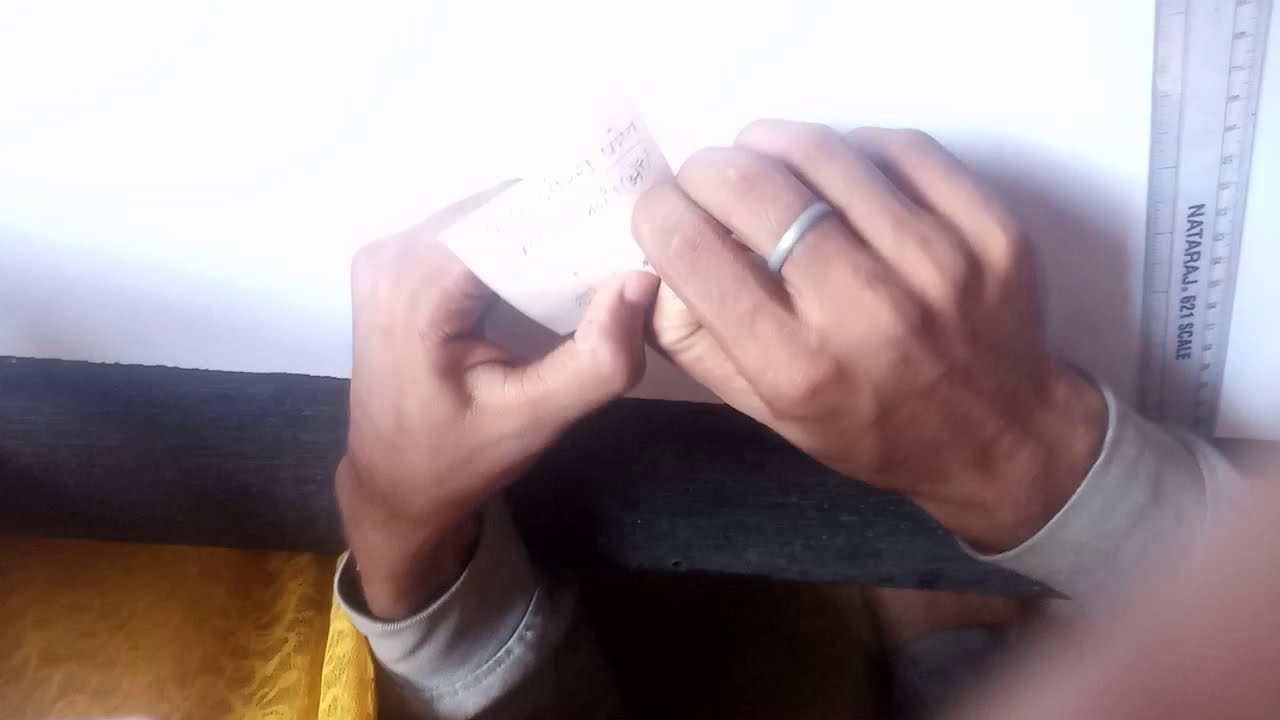The image captures a somewhat overexposed and blurry scene of a person working at a desk-like setup, possibly for drafting or art. The main focus is on the hands, which are positioned toward the left side of the frame. The right hand, adorned with a thin silver ring on the middle finger, is holding a white piece of paper with illegible writing and numbers, possibly betting slips. Both hands emerge from the cuffs of a white long-sleeve shirt, contrasted by black sleeves.

In the background, a white surface transitions from shadowed to completely overexposed, making it challenging to discern specific details. A clear plastic ruler labeled "Nataraj 621 Scale" lies vertically on the right side of this surface. The desk or table beneath the hands appears to have a dark wooden texture. Additionally, a black bar runs slightly tilted across the image from left to right, partially obscured by the hands. To the right of the hands, there is an indistinct scale with numbers, further adding to the mysterious and cluttered composition.